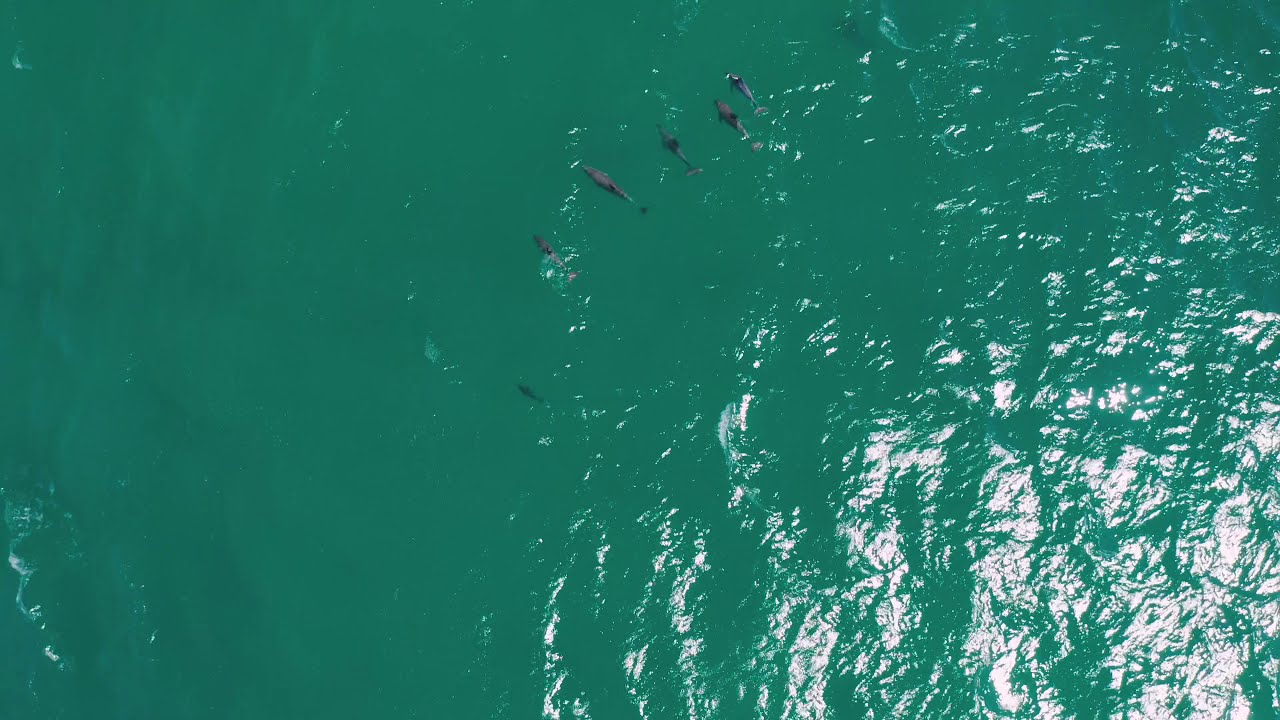This aerial photograph captures a serene moment in a large body of light green water, possibly the ocean. The sun casts its reflections, creating a brighter patch in the bottom right corner of the image, where gentle ripples can be seen. Approximately six or seven dolphins, though they could be mistaken for sharks, swim gracefully in a near-perfect line, progressing towards the upper left side of the frame. Their sleek, light-gray bodies contrast beautifully against the green water. Among them, one dolphin lags slightly behind and dives deeper beneath the surface. The others display varying levels of submersion; some are just beneath the surface with their fins exposed, while others are almost fully submerged. The dolphin furthest along the line appears lighter in color and reflects the sunlight differently, adding a touch of brilliance to the natural scene. The photograph’s perspective from above, likely captured by a drone, offers a breathtaking view of the aquatic formation.